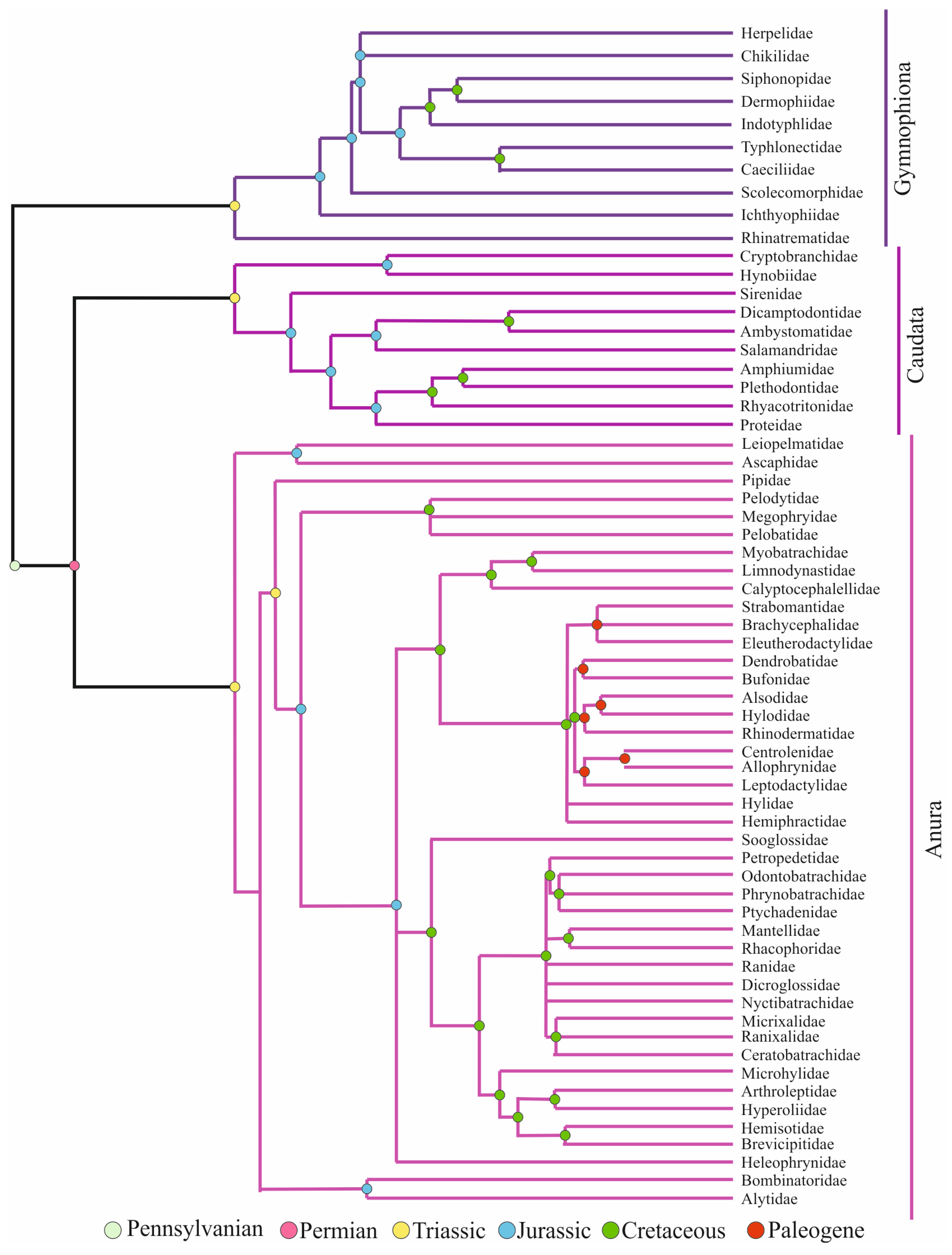The image presents a detailed horizontal chart that categorizes the families and subfamilies of various animals through genus connections, depicted with lines and dots in various colors. The chart, filled with specific Latin terminology, organizes these animals into three sections: Anura, Caudata, and Gymnophiona, each denoted by distinct colored lines—long pink lines, short purple lines, and longer dark purple lines, as well as some black lines showing interconnections.

The chart is color-coded to represent historical periods, with a legend at the bottom indicating the timeframes: Pennsylvanian (white dots), Permian (pink dots), Triassic (yellow dots), Jurassic (light blue dots), Cretaceous (green dots), and Paleogene (red dots). These colored dots are distributed throughout the chart, linking different animal genera to their corresponding periods, showing evolutionary branching from common ancestors and illustrating their interconnected relationships.